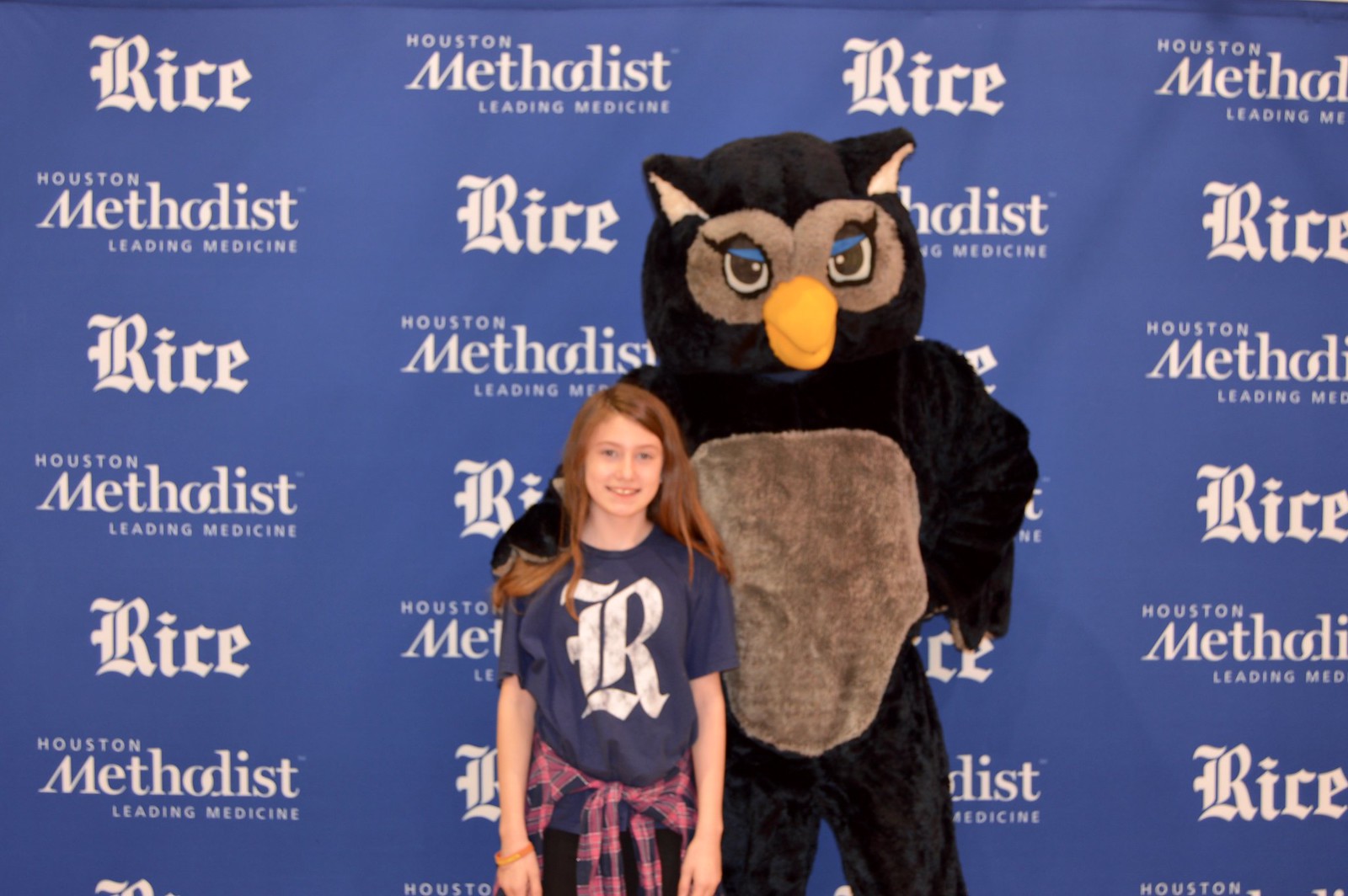The photograph captures a young Caucasian girl, around 10 to 12 years old, standing next to the Rice Owls mascot. She has long, straight hair that appears light brown or red, parted on the side, and she’s smiling brightly, revealing her upper row of teeth. She's dressed in a dark blue or purple short-sleeve shirt with a white Gothic-style "R" on the chest, likely representing Rice University. Around her waist, she has tied a pink and navy blue plaid long-sleeve shirt. 

The owl mascot standing to her right has a predominantly black costume with a brown belly, brown markings around its large eyes, brown inside its ears, and a yellow beak with blue eyelids or eyelashes. The mascot's right wing/arm is draped over the girl's shoulder. 

They are in front of a blue wall adorned with white, repeating text that alternates between "Rice" and "Houston Methodist Leading Medicine." This pattern creates a recognizable backdrop for the Rice University and Houston Methodist institutions. The photograph emphasizes a sense of joy and community spirit, captured in a realistic, representational style.